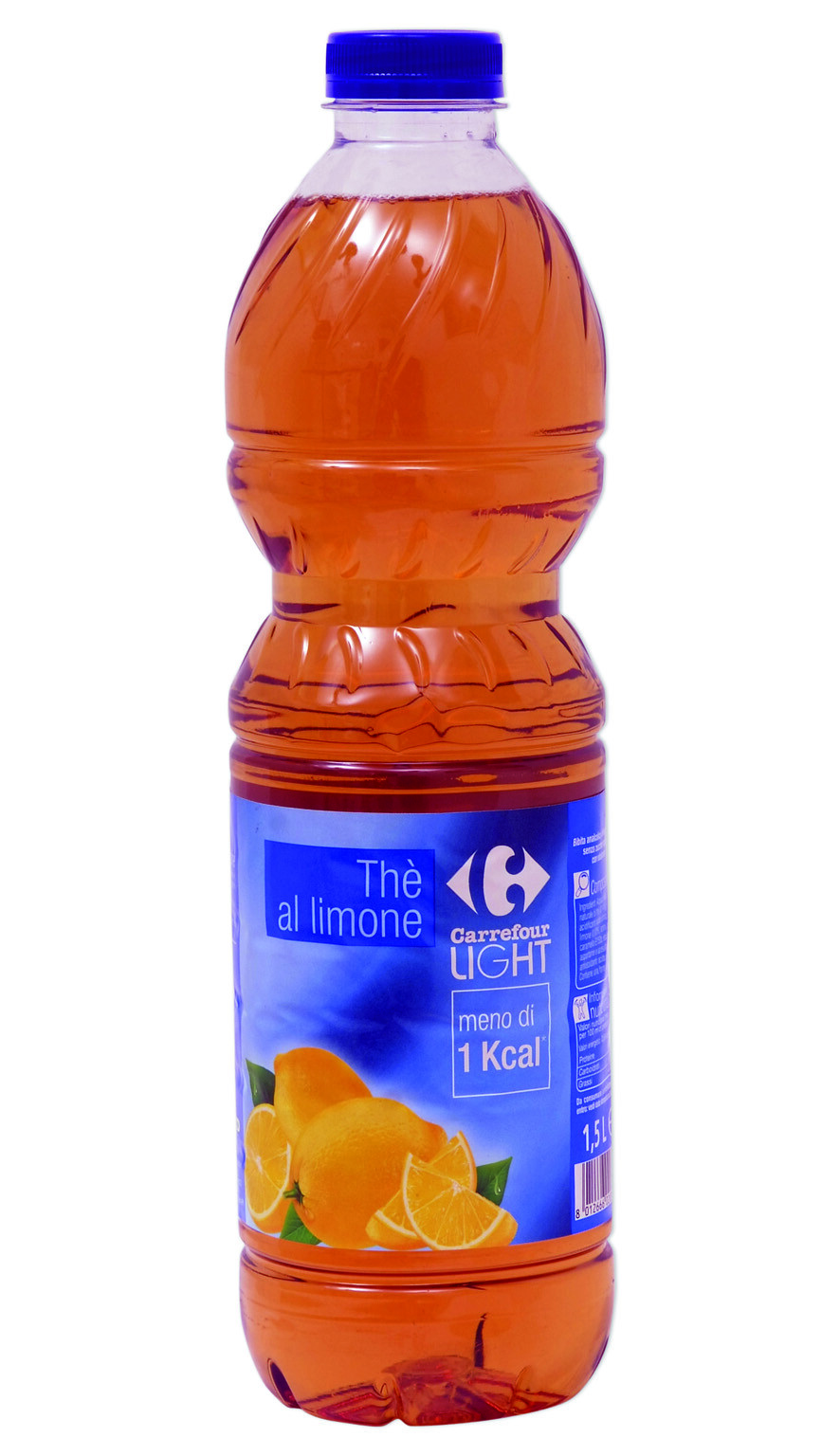The image is a photograph of a tall, clear plastic bottle filled with a light brown, amber-colored beverage. The bottle is topped with a blue screw cap, and it is set against a white background. The beverage inside appears to be lemon-flavored tea, as indicated by the label. 

The blue label, which covers the bottom half of the bottle, prominently features images of sliced lemons or possibly oranges, along with some green leaves. It has the word "Té" (T-H-E with an accent) followed by "al limone," suggesting the drink is lemon tea. The branding also includes the word "Carrefour" from the store it is sold at. 

Additionally, the label states that the beverage is "light," implying it is a diet drink, with "meno di 1 Kcal" written underneath, indicating it contains less than one kilocalorie. The far right edge of the label appears to include additional information and a partial barcode, although these details are not fully visible in the image. The bottle's slight narrowing above the label provides a comfortable grip for holding.